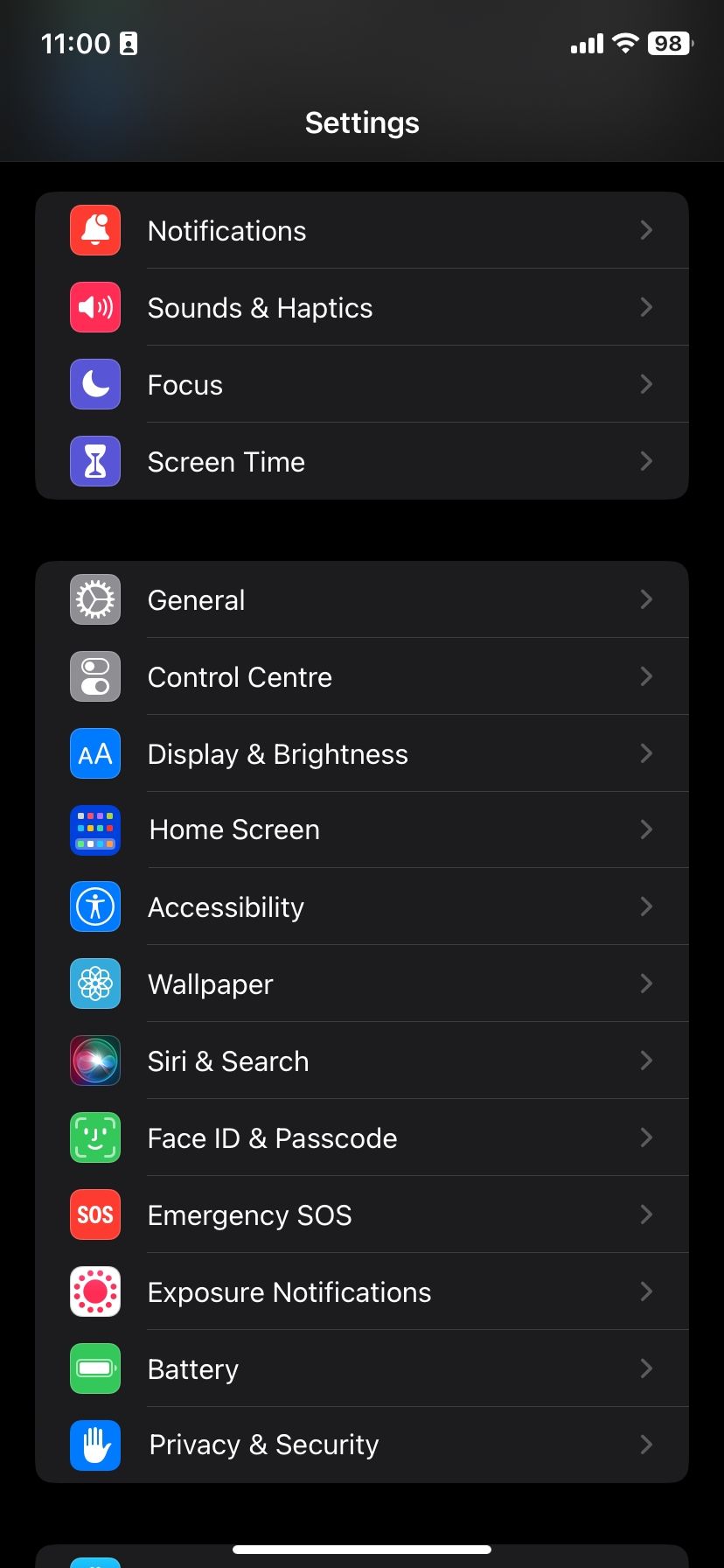This image is a screenshot from a smartphone with a black background. In the upper left-hand corner, "11:00" is displayed in a white font, indicating the time. On the upper right-hand corner, there is a battery icon showing a 98% charge, along with the Wi-Fi and cellular connection icons, all in white.

Central to the screenshot is the word "Settings" in white font, indicating the currently selected menu. Below "Settings," there's a vertical list of system options, each accompanied by a corresponding icon to its left. The list includes (from top to bottom):

1. Notifications
2. Sounds & Haptics
3. Focus
4. Screen Time
5. General
6. Control Center
7. Display & Brightness
8. Home Screen
9. Accessibility
10. Wallpaper
11. Siri & Search
12. Face ID & Passcode
13. Emergency SOS
14. Exposure Notifications
15. Battery
16. Privacy & Security

Each option is labeled in white font, and the left-side icons are distinct and colorful. Notably, some icons are red, others are purple, a few are various shades of blue, and two are silver. The icons provide a visual cue for each setting category, enhancing the usability and aesthetic of the settings menu.